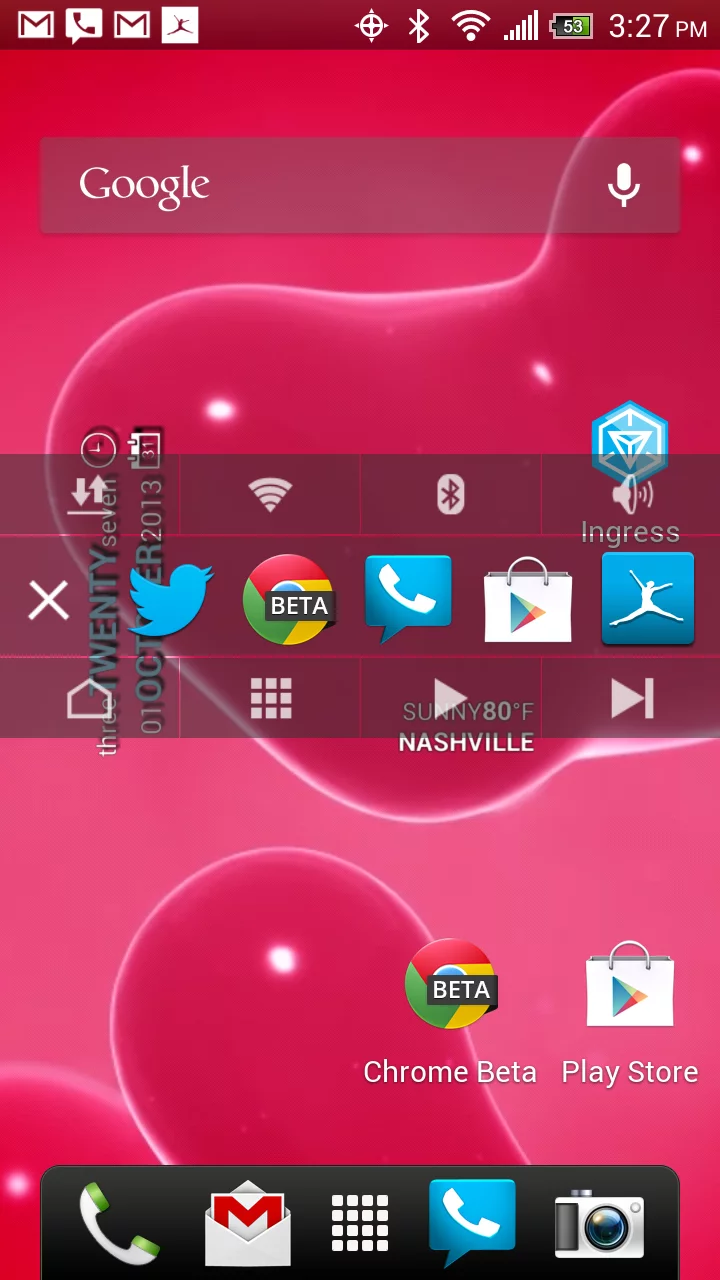The image displays a vibrant background transitioning from red at the top to pink at the bottom. The header features a burgundy banner with multiple icons inside squares: an 'M', a telephone, another 'M', and an icon of a leaping person. Below this section, the status bar shows various indicators - a Bluetooth icon with a battery level at 53%, WiFi signal, cell signal strength, and the time of 3:27 PM.

The main section presents a pink background adorned with scattered red blobs. Prominently placed is a search bar with the word "Google" in capitalized white letters. To the left inside this bar is a capital 'G', while on the right side is a white microphone icon. Beneath this bar, a darker banner hosts several social media and utility icons: Twitter, a phone, Chrome, a shopping cart, and another blue square with a leaping person, reminiscent of a gymnast.

Towards the bottom, there is a section labeled "Beta" next to the Chrome browser and Play Store icons. The footer contains additional icons for phone, email, camera, and another phone symbol against a blue background.